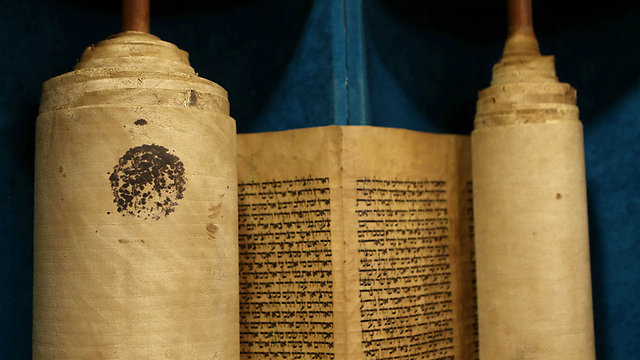The image depicts an ancient scroll displayed in a museum setting, carefully presented within a velvety blue holder. The scroll is unrolled in the center, showcasing intricate Arabic manuscript writing on aged, delicate paper. This paper, reminiscent of traditional ancient papermaking techniques, highlights the historical significance of the artifact. The scroll is anchored by two vertical wooden rods, one on each end, with the left side appearing thicker due to the wound-up portion of the scroll. An orange hue characterizes the wooden rods, adding a contrasting element to the overall presentation. A distinctive black marker is visible on the left side of the scroll, further emphasizing its historical importance and meticulous preservation.